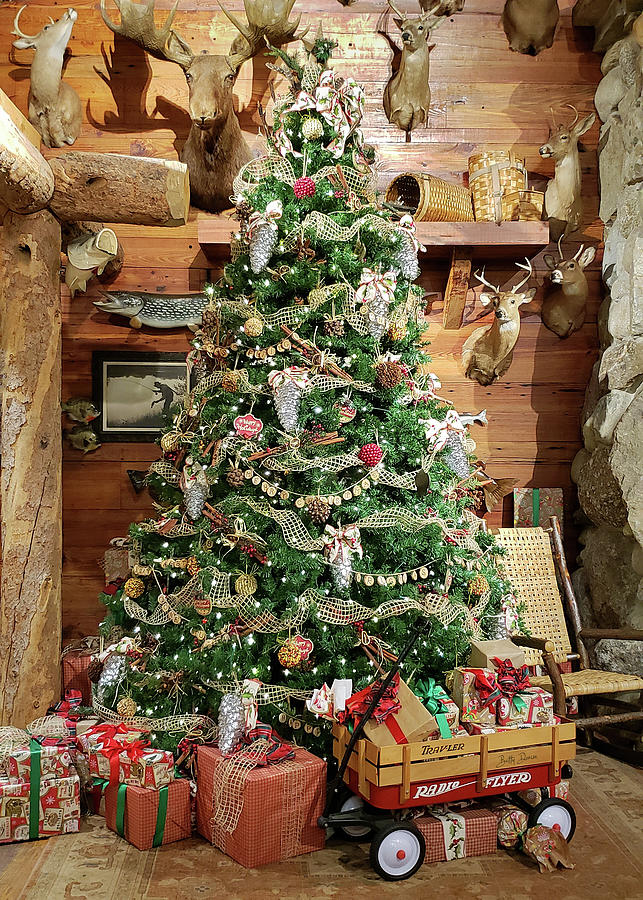In the center of the image stands a beautifully decorated Christmas tree, tall and green, adorned with gold ribbon garlands, strings of coins, and a variety of ornaments. Scattered among the branches are silver and brown pinecones, as well as clusters of red berries, all contributing to its festive charm. Topping the tree is a large, elegant bow. In front of the tree, a red Radio Flyer wagon brimming with gifts is prominently displayed, with additional presents wrapped in red and white paper scattered on the floor around it.

The setting is a cozy, rustic log cabin, its walls lined with horizontal orangey wood slats and accented with large wooden beams and stone. Mounted on the walls are several deer heads, a moose, and some fish, adding to the cabin's mountain appeal. A wooden chair with a wicker seat sits next to the tree, enhancing the homey atmosphere. Above, shelves hold Longaberger baskets, contributing to the scene's quaint, traditional vibe. A lone photograph of a man fishing hangs on the wall, further encapsulating the cabin’s rustic charm.